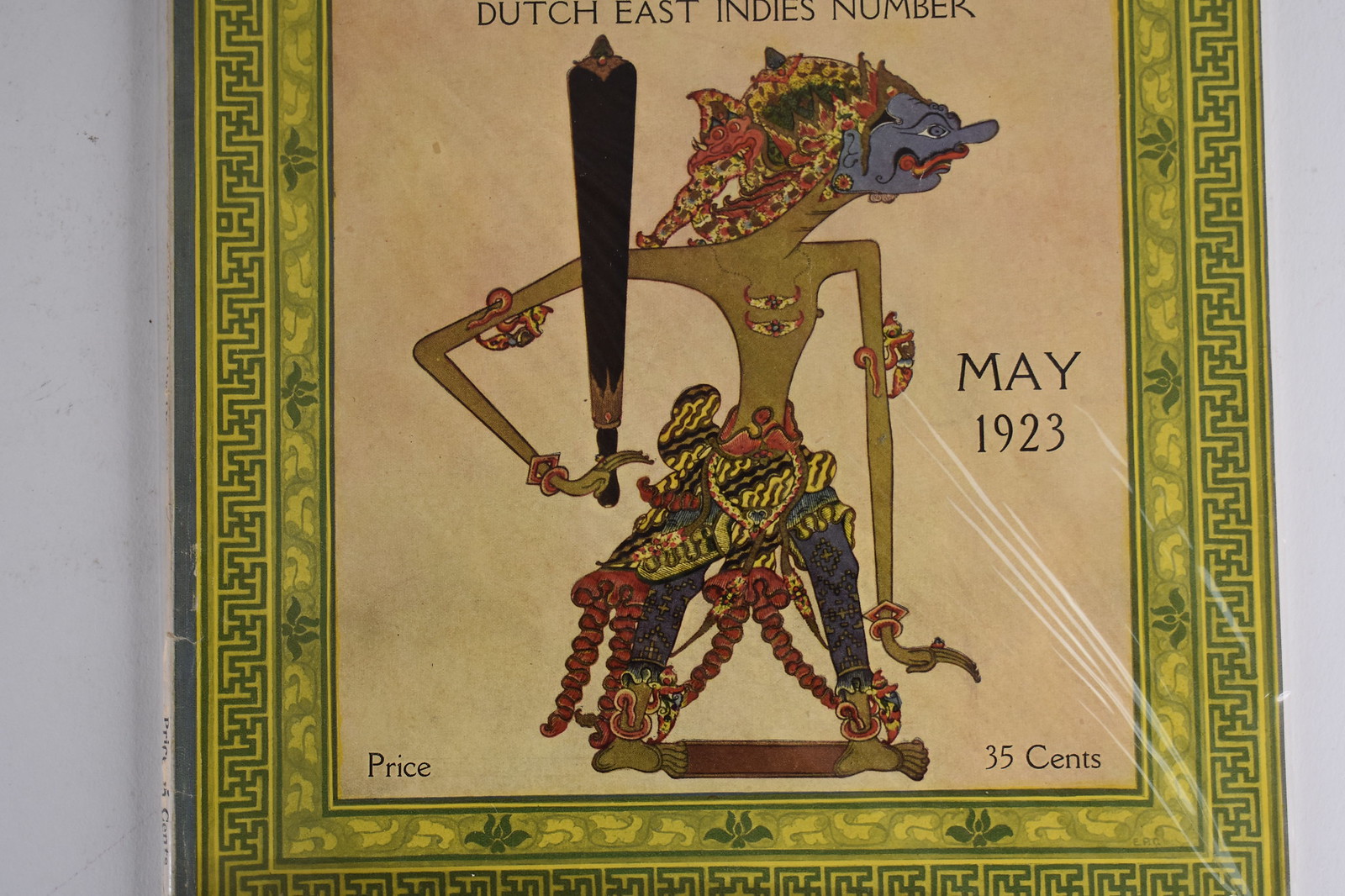This landscape-oriented color photograph captures a vintage framed stamp from May 1923, believed to depict a piece of detailed artwork representative of the Dutch East Indies. The central figure in the image is a unique, anthropomorphic character with an elongated neck and a narrow chest and stomach. Its face is distinctly blue, contrasting with its brown body. Adorning the character is a colorful, intricate headdress composed of red, yellow, and green hues, complemented by blue pants intricately designed with additional accessories. The figure holds a black baseball-like bat in its right hand and is embellished with banded bracelets on its upper arms and multiple decorative belts around the waist. The feet are adorned with ankle bracelets, maintaining a joined stance. The backdrop of the stamp is a beige cream color, framed with a decorative Greek design in dark green and flourishes of cream, featuring two bands. The border adds to the intricate aesthetic with its gold hue. Text on the stamp includes "Dutch East Indies number" at the top and "35 cents" at the bottom right corner. The painting itself is affixed to a light blue wall and might be under plastic, as suggested by visible streaks, enhancing its preservation and showcasing its artistic and historical value.